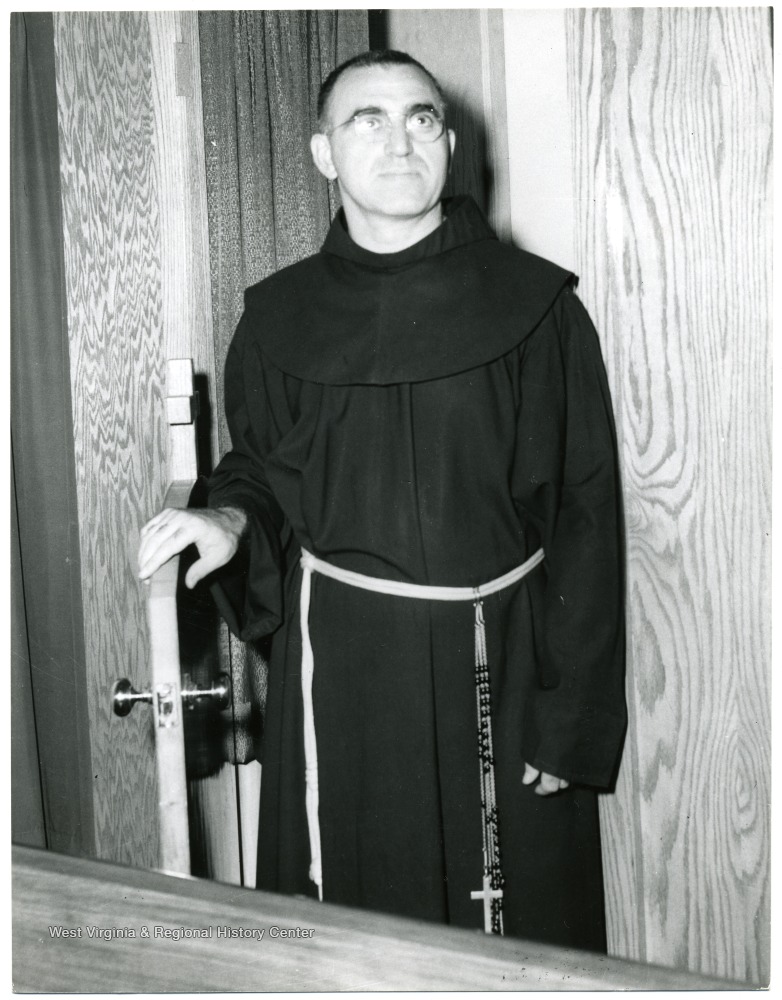The black and white photograph depicts a Catholic priest standing next to a heavily grained wooden wall. He is wearing a long black robe with a white string belt, from which hang rosary beads and a cross. The priest, who has a short buzzed haircut and glasses, gazes upwards while holding open a small half door, possibly leading to a baptism room with a viewing tub. Behind him, a dark curtain is partially visible, and a wooden table occupies the bottom left corner of the image. Overlaying the bottom left is the text "West Virginia Regional History Center."